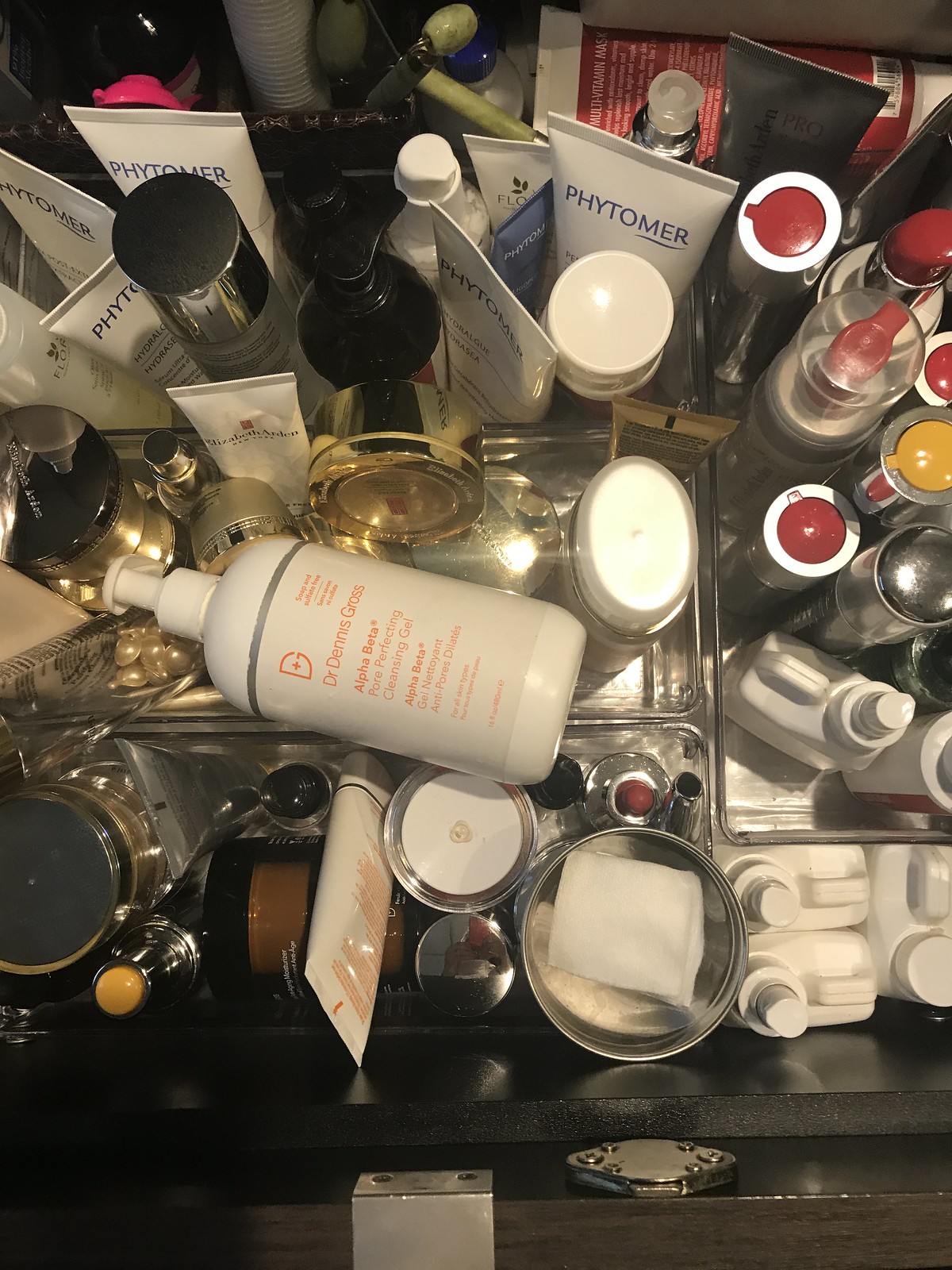This photograph captures a cluttered indoor scene with a variety of skincare and makeup products scattered across a surface. The assortment includes numerous plastic dispensers and spray bottles, featuring an array of colors such as white, red, yellow, pink, and brown. The containers vary greatly in size and shape, adding to the visual interest of the image. The lighting in the setting is dim yet sufficient to clearly identify the different products. The overall composition is framed within a square rectangle, providing a compact and detailed view of the disorganized array of beauty items.